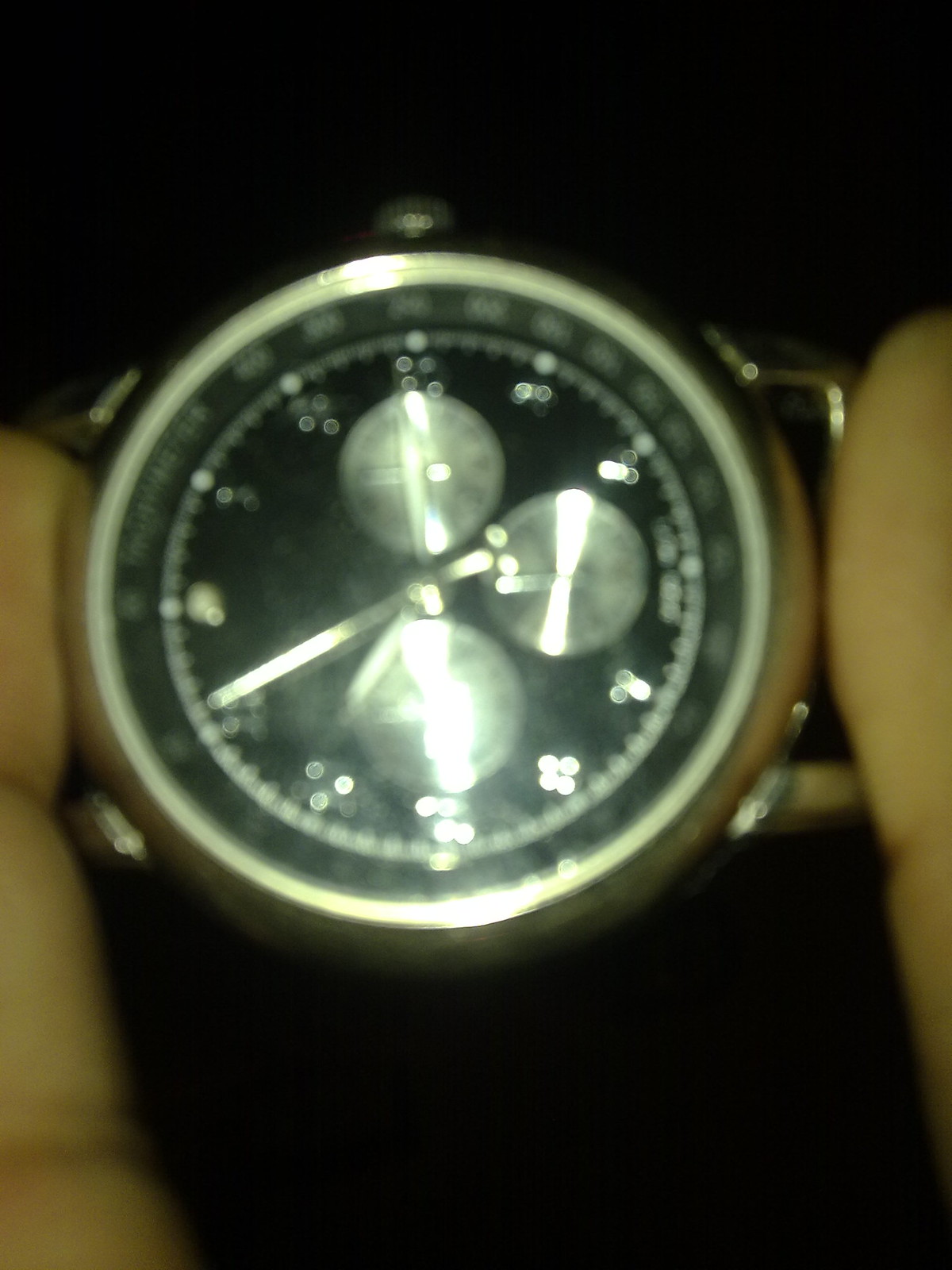In this image, a close-up view captures two fingers—specifically the thumb and index finger—pinching and holding a wristwatch by its top and bottom edges. The focal point of the wristwatch is its face, which is characterized by a sleek, black base. The watch hands, crafted from a striking silver, stand out against the dark background, offering a sharp contrast. On the lower part of the watch face, three small, shiny dials, also in silver, can be seen. These dials catch and reflect the light, giving them a lustrous, illuminated appearance. Encircling the watch face is a polished silver border that adds a touch of elegance. The watchcase itself is a rich, dark brown, complementing the overall design. The background of the image is uniformly black and dark, ensuring that the wristwatch is the primary focus of the viewer's attention. The fingers holding the watch are positioned in a way that highlights the fine details of the timepiece, which is suspended against the dark backdrop.